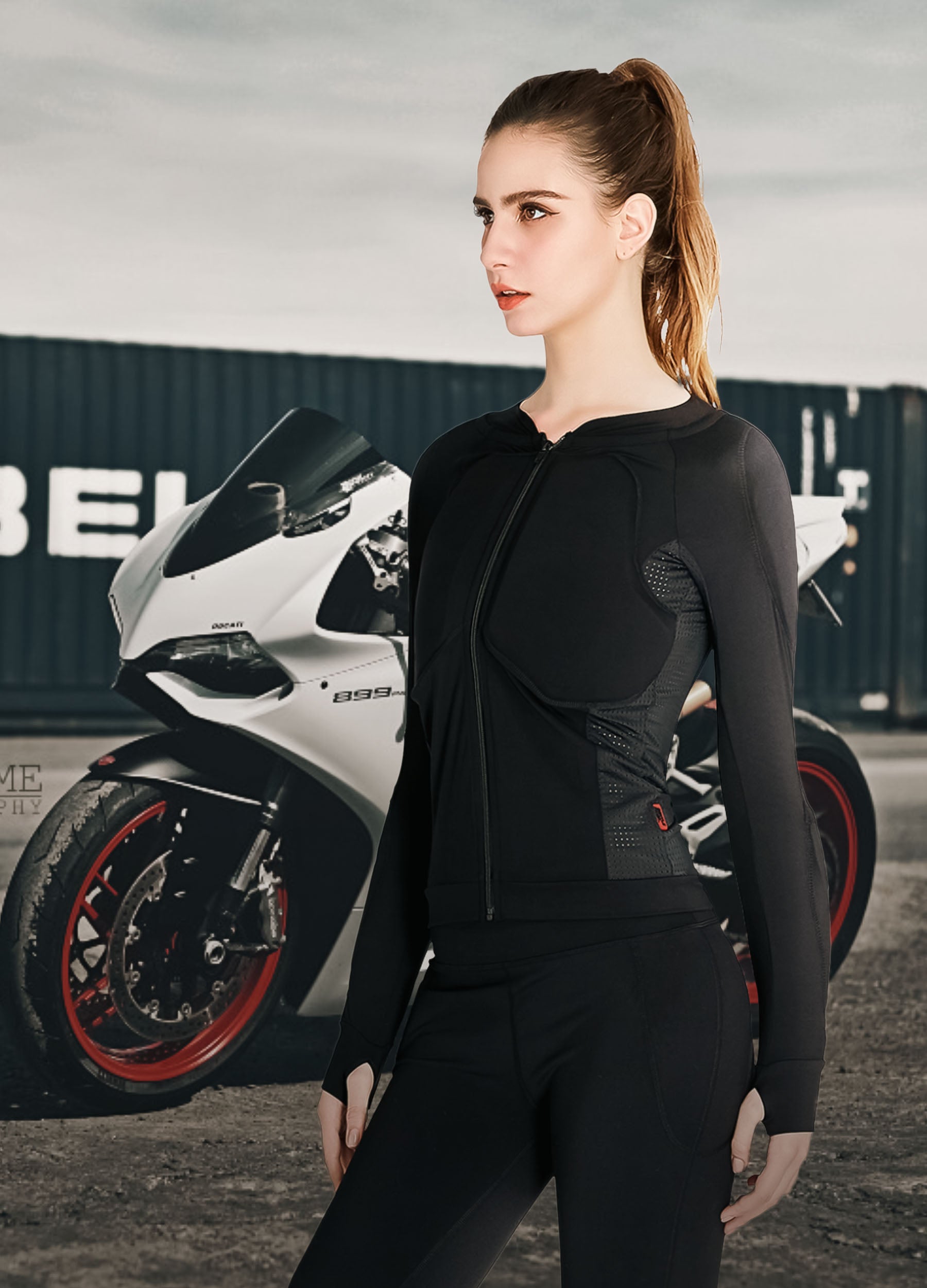The image features a young, white-skinned woman with brown hair pulled back into a ponytail, modeling motorcycle gear. Her hair, darker at the roots and lighter, almost dirty blonde, in the ponytail, adds a striking contrast to her look. She is wearing a form-fitting, black, padded jacket with a full zipper in the middle and thumb holes at the sleeves' ends. The jacket has gray breathable panels under the arms with small perforations revealing a white lining, and a small orange tag along the side seam. Her pants are black and similarly styled, with noticeable pads on the hips. 

The woman is posed standing front-facing but slightly turned to her left, with her hands at her sides. Her gaze is directed to the left, and she sports red lipstick. The backdrop showcases a white Ducati-style sports motorcycle with the number 899 on it, featuring wheels that have a red trim. Further behind, there is a greenish shipping container with partially visible white lettering "BE" and "LI." The setting appears overcast with a cloudy gray sky, contributing to the impression that the woman might be superimposed onto the background, as her legs from the knees down are cut off in the image.